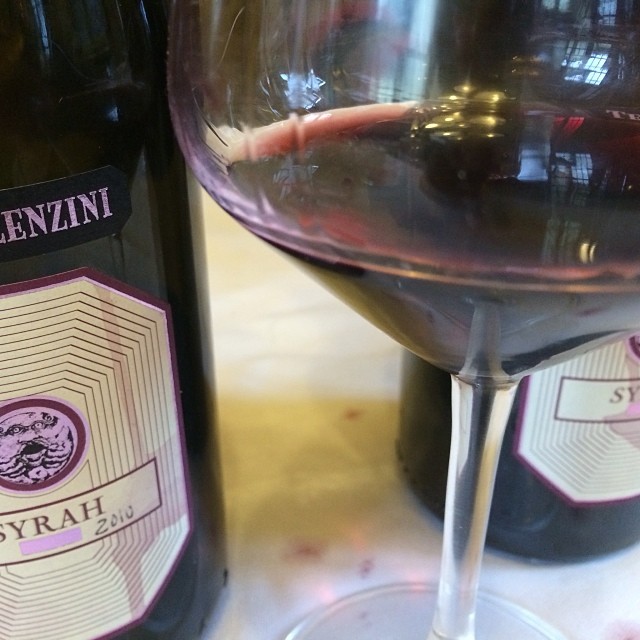This close-up image features a crystal-clear, long-stemmed wine glass partially filled with dark red wine, positioned on a white table. Flanking the glass are two wine bottles, though only one is distinctly visible on the left-hand side. The bottle displays a half-visible brand name, showing the letters "E-N-Z-I-N-I." The bottle's label, predominantly beige, features a detailed and somewhat peculiar design: an octagonal pattern containing the illustrated face of a man with hands gripping his mouth. The label also prominently reads "SYRAH" and indicates the wine is from the year 2010. The wine within the bottle is described as having a dark purple hue.